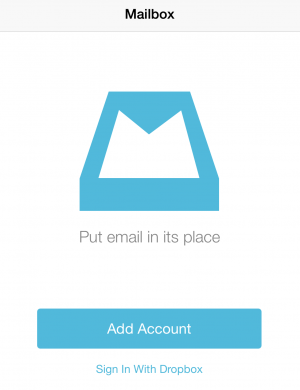In this screenshot set against a solid white background, there is a prominent light gray banner spanning horizontally across the top of the screen. Centered within this banner, in bold black text, is the word "Mailbox." Directly below this banner, there is a stylized icon depicting a piece of mail, rendered in shades of blue and white. Beneath this icon, a caption in light gray text reads, "Put email in its place." Following this line of text, there is a light blue action button with the phrase "Add Account" inscribed in white text. At the bottom of the screen, there is another piece of text in light blue reading "Sign in with Dropbox."